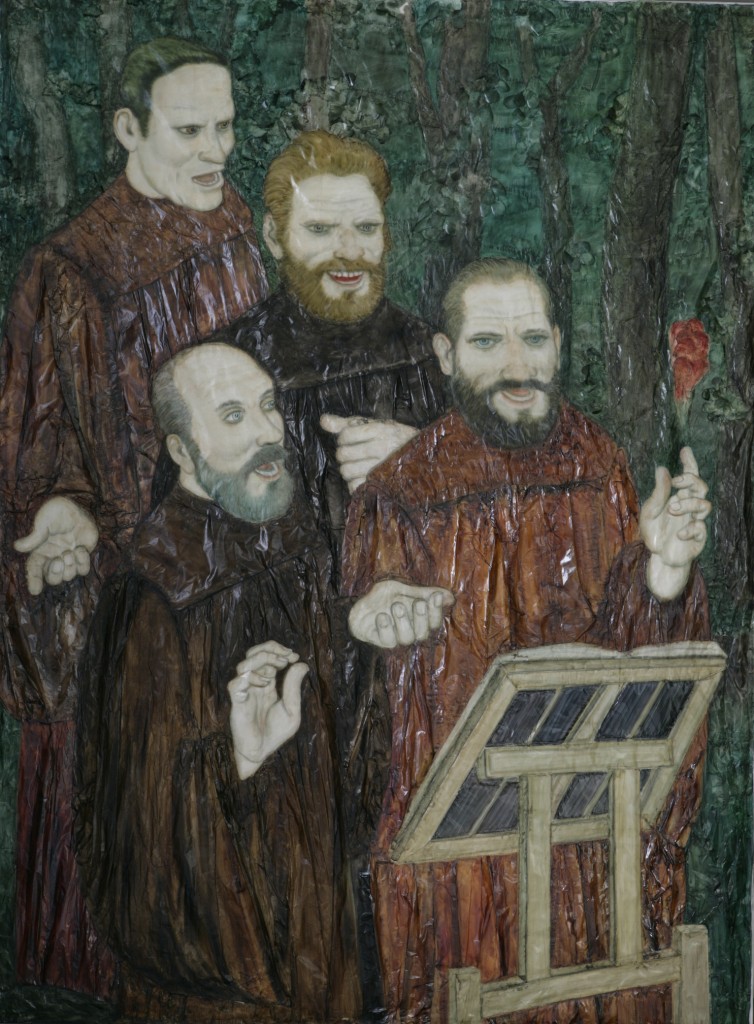In this detailed and textured painting, four men dressed in robes are gathered around a small wooden podium in the lower right corner, likely containing a music book or sheet. These men appear to be singing, their expressions ranging from smirking to joyous, suggesting they are enjoying themselves. From left to right, the figures display a variety of looks: one man, wearing a brownish cloak, is balding with a gray beard and mustache. Another man, clad in a dark gown and standing behind the podium, has red hair, a red beard, and a red mustache. Next, a man in the forefront of the image, also with a beard and mustache, possesses brown hair and is distinguishable by the red flower or possibly a catalily he holds in his left hand. The remaining singer, positioned behind the others, is a white man with dark side-parted hair, distinguished by his clear lack of facial hair. This scene unfolds against a dark green, stone-like background, giving the image a distinctly focused and intimate feel, as if capturing a private moment of rehearsal or performance by what seems to be a quartet.